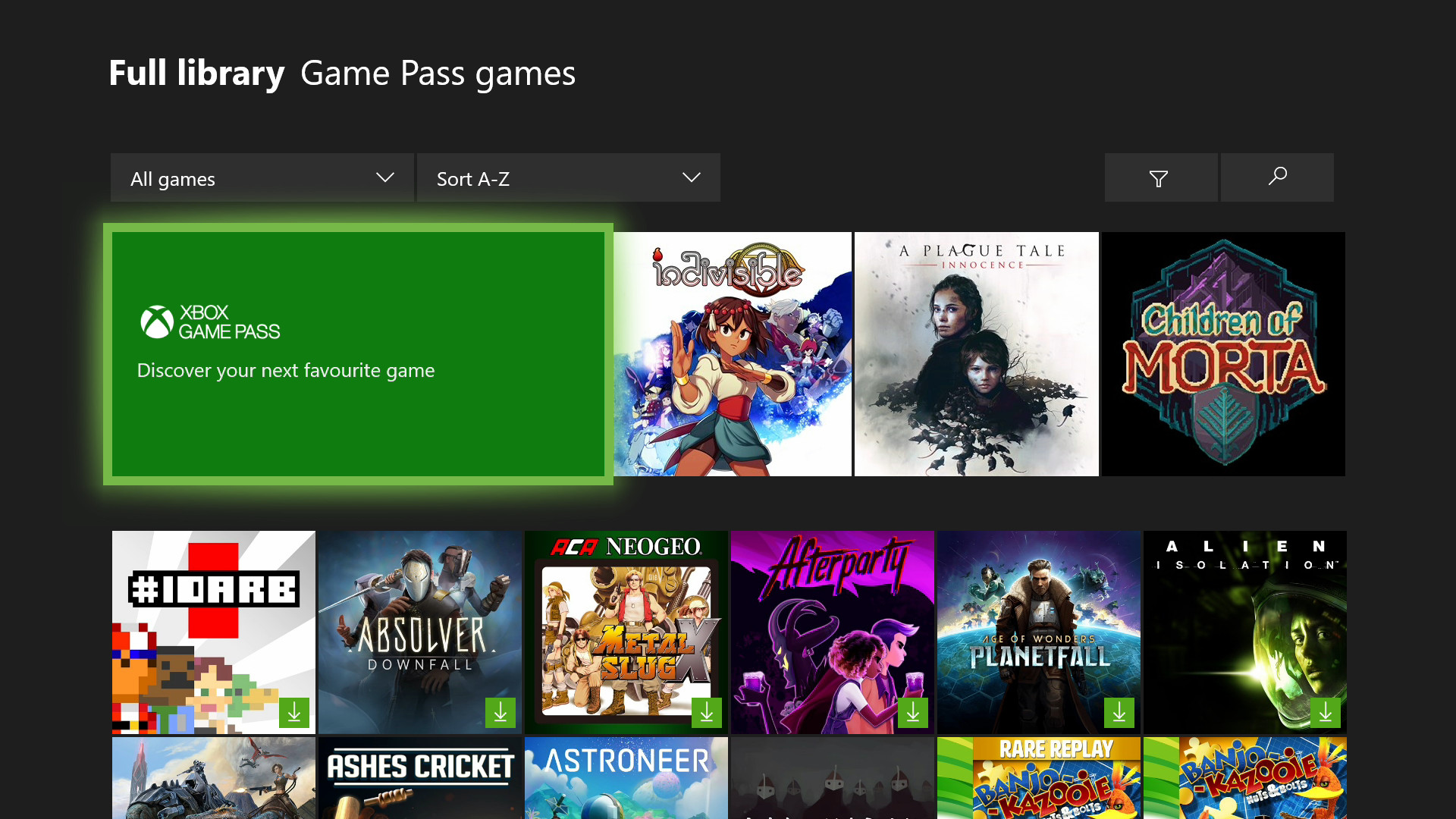This image is a screenshot taken from a gaming website, specifically showcasing the Xbox Game Pass library. The overall background is black, giving it a sleek and modern appearance. At the top of the page, bold white text reads "Full Library Game Pass Games." Just below this, a navigation bar includes an option labeled "All Games," allowing users to browse the entire collection. Additionally, there are dropdown menus for sorting options, such as "Sort A to Z," which help users find specific games more easily.

On the left-hand side of the page, towards the bottom, there is a prominent green box with a darker green center and a lighter green border. This box contains marketing text that reads, "Xbox Game Pass: Discover your next favourite games," notably using the British spelling of 'favourite' with "F-A-V-O-U-R-I-T-E."

Below this section, the page displays a vertical list of game titles available on Xbox Game Pass, starting with:

- **Invisible**
- **A Plague Tale**
- **Children of Morta**
- **#IDare**
- **Absolver: Downfall**
- **Neo Geo**
- **Afterparty**
- **Planetfall**
- **Alien**

The list continues beyond what is visible in the screenshot, suggesting a diverse and extensive catalog of games for users to explore.